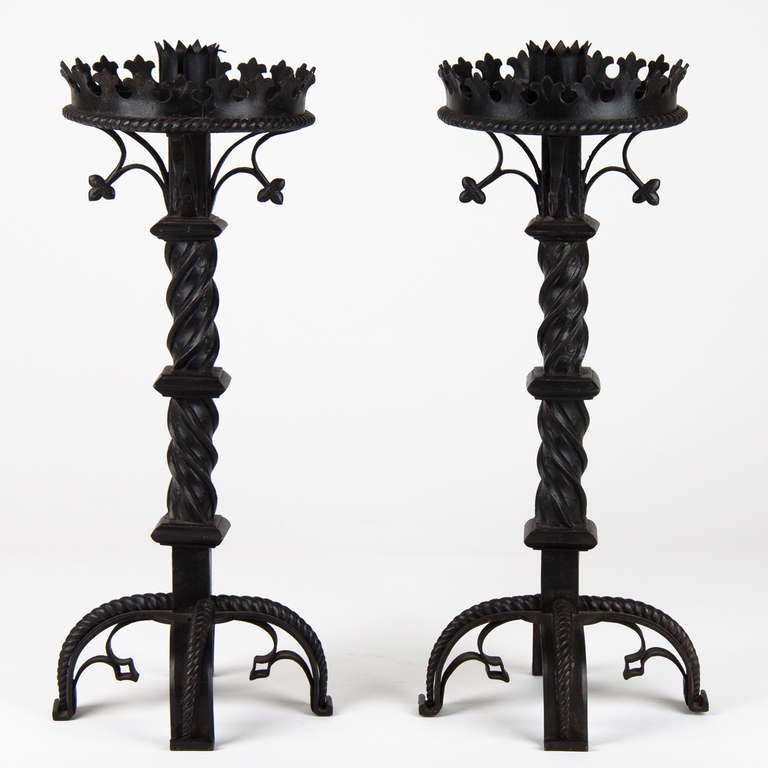This photograph showcases two identical black wrought iron stands set against a seamless, pure white background, creating a clean and modern look. The stands, possibly used for either candles or plants, exhibit an intricate and decorative design. Each has a sturdy four-pronged base adorned with ornate details, providing both stability and a touch of elegance. Rising from the bases, the stands feature a twisted, rope-like neck that adds a dynamic, sculptural element to their vertical structure. The top of each stand is circular with a beveled edge, resembling a flat crown that seamlessly transitions into a pointed, crown-like holder where a candle or plant might be placed. The overall intricate ironwork of the stands, with its combination of twirls and elaborate design elements, highlights their elaborate craftsmanship and refined aesthetic.